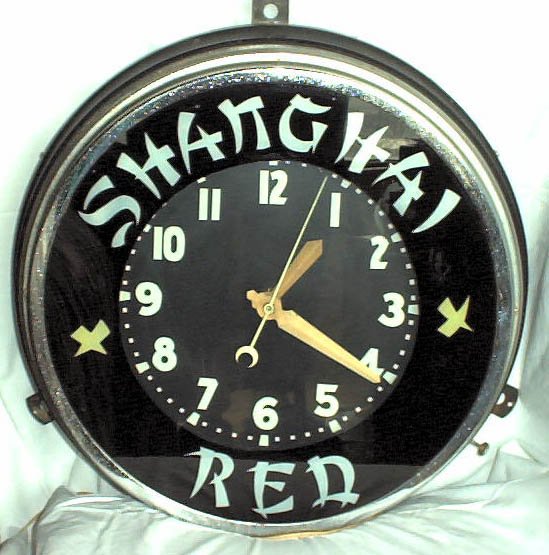In this square color photograph, the focal point is an artistic-looking, round pocket watch with a glass-like face. The backdrop comprises a piece of fabric with visible wrinkles that has been overexposed, casting a bright background. The metallic watch features a detailed dial, prominently marked with 12 white numbers and adorned with gold minute, second, and hour hands. The hands’ intricate designs include a thin microsecond hand with a crescent moon at its end.

The dial's black background is accented by reflective surfaces, with "Shanghai" inscribed at the top in an Asian-style font, and "Red" written below. Flanking the central face are indications of yellow birds or possibly ornamental marks. The circumference of the watch has a metal edge with a notable hole at the top, likely for hanging, and a winding knob protruding from the lower right-hand side at the back. The watch is not attached to any chain, suggesting it is meant to be carried as a standalone timepiece.